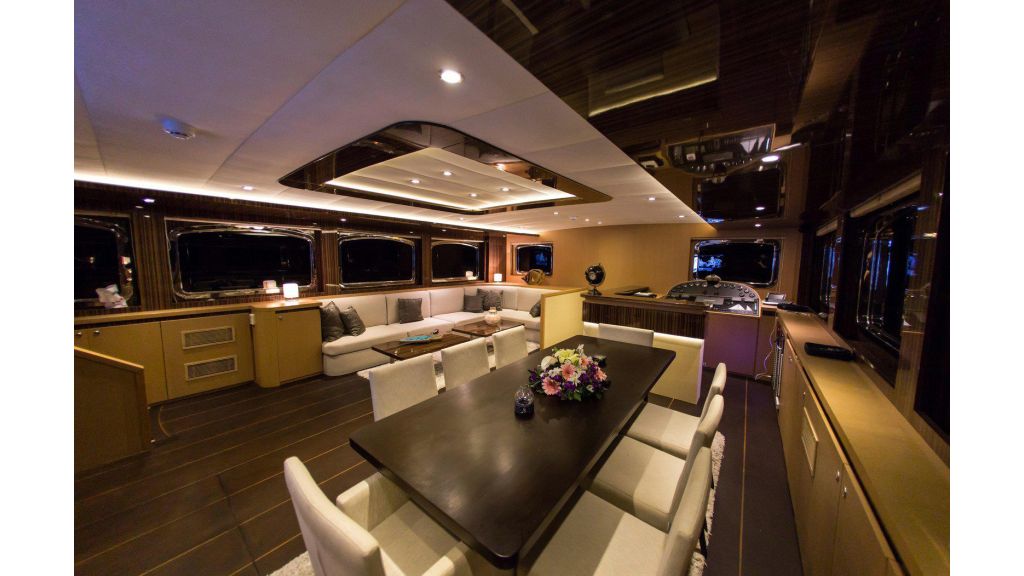This color photograph captures the luxurious interior of a grand yacht dinette area from a right-angle perspective. Dominating the foreground is an elegant, mahogany-hued dining table, adorned with a vibrant flower bouquet. The table is surrounded by eight white-cushioned chairs—three on each of the longer sides and one at each end. Framing this opulent setting are sleek, wooden cabinets lining the walls. Above these cabinets, long, rectangular windows framed in silver metal provide ample natural light and stunning views. 

The yacht boasts a pristine white ceiling with recessed lights that enhance the ambiance. The flooring, reminiscent of polished wood planking, furthers the nautical theme. In the rear, an L-shaped white couch with gray pillows invites relaxation, and a subtly integrated control panel with a window next to it hints at the vessel’s sophisticated navigation technology. Though partially obscured, a large screen TV or desk area is visible in the distance, completing this image of plush maritime elegance.